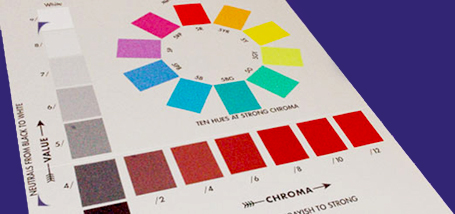This photograph features a white color chart set against a dark blue background. The chart is oriented diagonally from the top left to the bottom right. Dominating the upper section of the chart is a circular color wheel displaying a spectrum of colors arranged clockwise: starting with red, transitioning through orange, yellow, light green, teal, different shades of blue, purple, pink, and returning to red. 

Beneath the color wheel, there are eight horizontally aligned, square color panels that transition from dark gray to various shades of red, eventually ending in lighter orange. Each panel has a black printed number beneath it, corresponding to different F-stops, but the numbers are too small to read clearly.

On the left side of the color wheel, there is a vertical gradient from white to gray rectangles, indicating a shift from less white to more gray and grainy textures. This gradient is accompanied by black text, which is too small to decipher, running perpendicularly along the stack.

At the bottom, aligned horizontally with the red-to-orange squares, is the word "Chroma" in black text, accompanied by an arrow pointing to the right. This detailed arrangement suggests the chart might be used for calibrating colors in photography or visual design.